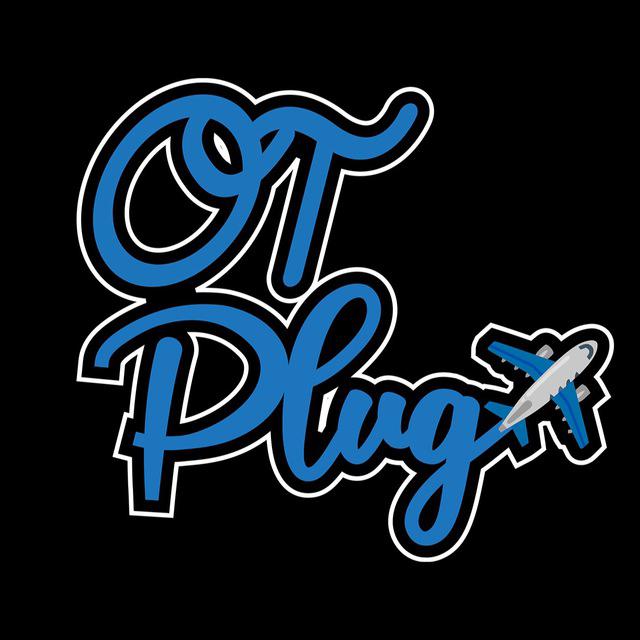The image features a stylish logo against a plain black background. The logo showcases the text "OT Plug" in bold cursive script, with "OT" appearing in capital letters above "Plug," which is written with a capital "P" followed by lowercase "l-u-g." The letters are primarily royal blue, outlined meticulously in black and layered with a white border for added contrast. Extending from the tail of the cursive "G" in "Plug," there is a detailed depiction of a cartoon-style jumbo jet airplane. This airplane has a white fuselage complemented by blue wings and tail fins, along with gray engines. Both the logo and the airplane feature the same tri-color outline of black and white, harmonizing the entire graphic art.